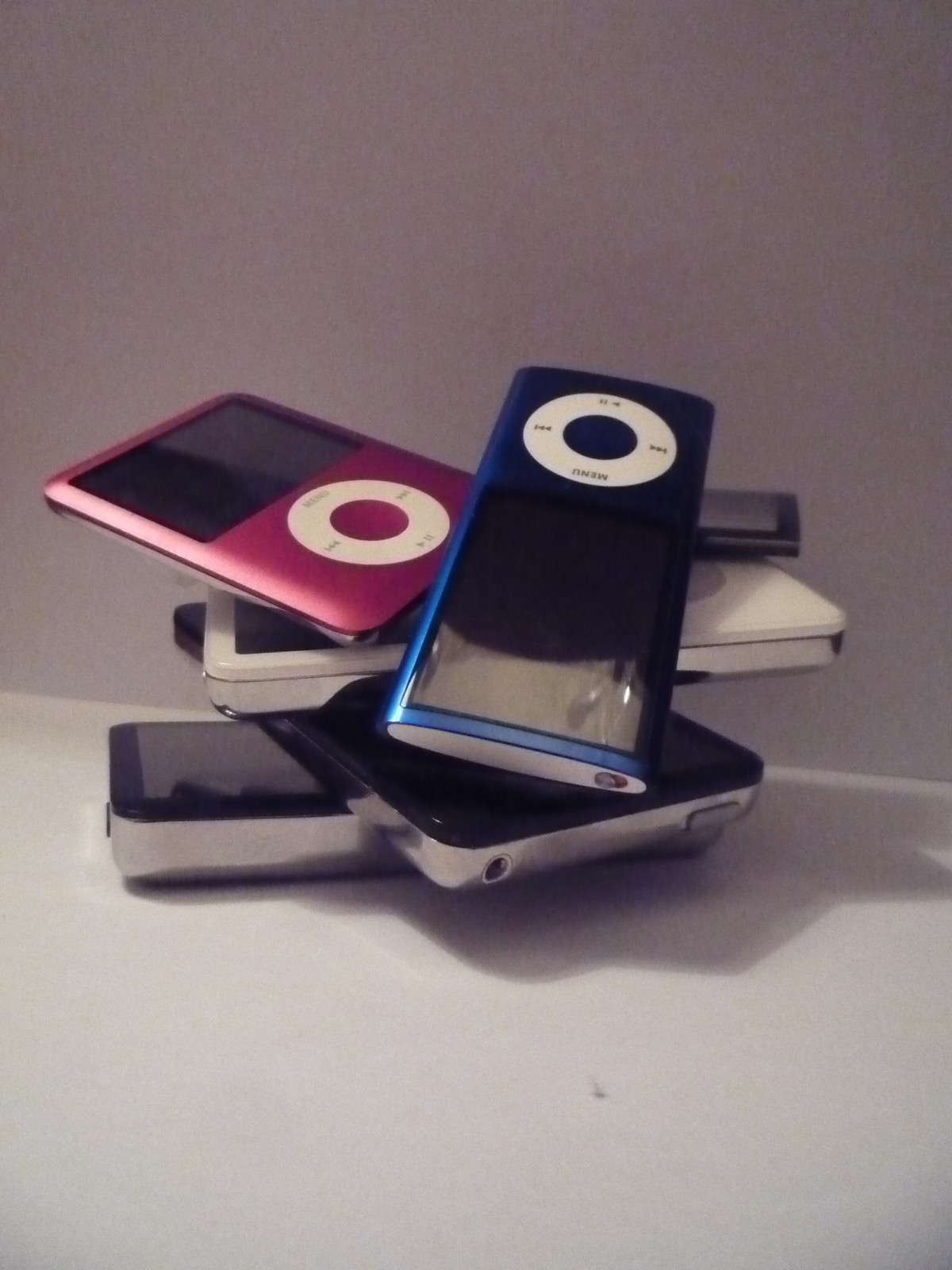In this indoor photograph, a stack of six colorful MP3 players, reminiscent of older iPods, is the focal point. Arranged haphazardly, the devices precariously balance atop a flat, grayish-white surface that matches the subtle background wall. The topmost player is blue, featuring a black screen and a distinctive white dial. Just beneath it, a red MP3 player with similar features lies askew. The stack continues with a white device followed by two silver and black players, each showcasing minor variations in color. The careful, possibly adhesive-assisted arrangement of these outdated gadgets creates a sense of impending collapse, emphasizing their central role amid an otherwise minimalistic setting.